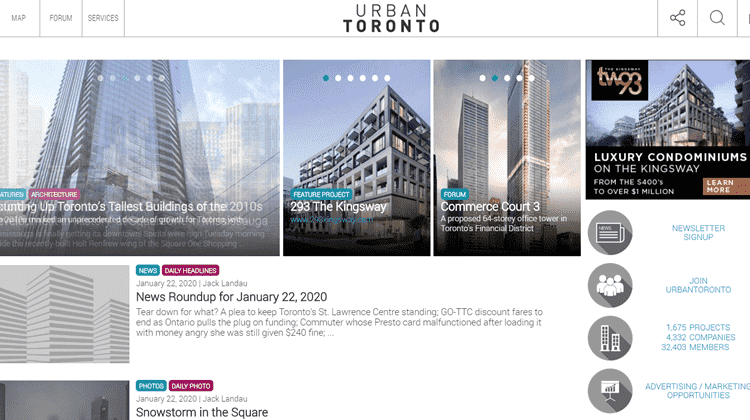The image showcases the homepage of a website dedicated to urban development and architecture in Toronto. At the top, the website's name "Urban Toronto" is prominently displayed in black. A navigation bar on the left features three menu options: "Map," "Forum," and "Services," while the right side houses a magnifying glass icon for search functionality and an icon with three dots for additional options.

Below the navigation bar, the page is filled with images of various buildings, each accompanied by descriptive text. One prominent image to the left highlights a project titled "293 The Kingsway," labeled as a featured project. Adjacent to it, another image introduces "Forum Commerce Court 3," a proposed 64-story office tower in Toronto's financial district. On the right, an advertisement showcases "TW 93 Luxury Condominiums on The Kingsway," with price ranges from $400,000 to over a million, and includes a button to learn more.

Further down, the page encourages users to sign up for a newsletter and join the Urban Toronto community, boasting 1,675 products, 4,333 companies, and 32,000 members. It also offers advertising and marketing opportunities.

On the left side, the page features recent articles, including a "News Roundup for January 22nd, 2020," and another piece titled "Snowstorm in the Square."